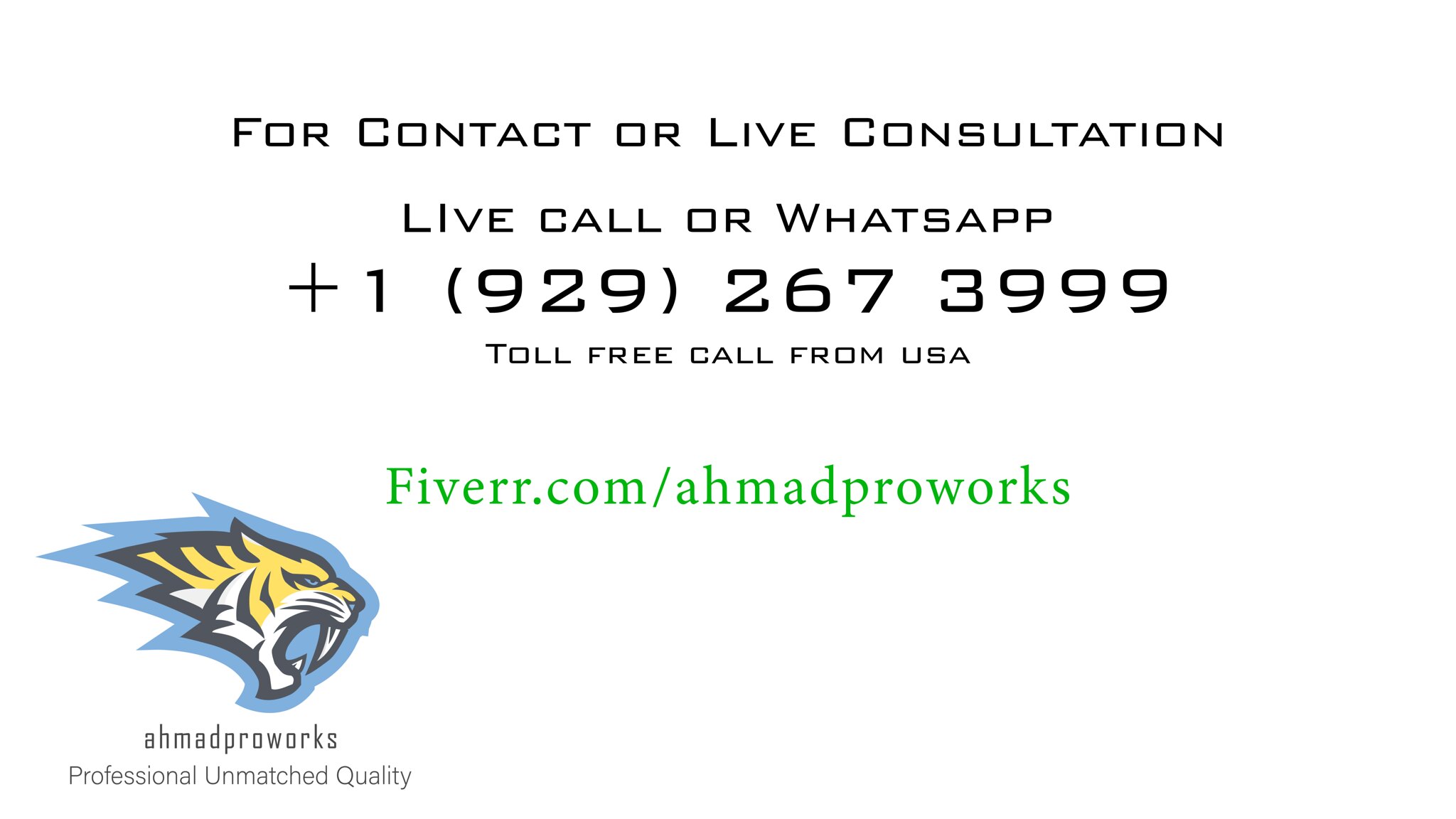The image is a wide rectangular digital advertisement with a white background. At the top, in bold black capital letters, it reads: "FOR CONTACT OR LIVE CONSULTATION". Directly below in gray text, it says: "Live Call or WhatsApp" followed by the phone number "1-929-267-3999" and the note "Toll Free Call from USA". In the center of the image, the website is prominently displayed in green font as "FIVERR.COM/AhmadProWorks". In the bottom left-hand corner, there is a detailed logo of a tiger's head with yellow and white fur, large white teeth, and traced in light blue. Below the logo, in black font, it reads: "Ahmad Pro Works" and beneath that, the phrase "Professional Unmatched Quality". The overall color scheme is primarily black, gray, and green with the tiger logo adding a touch of color.